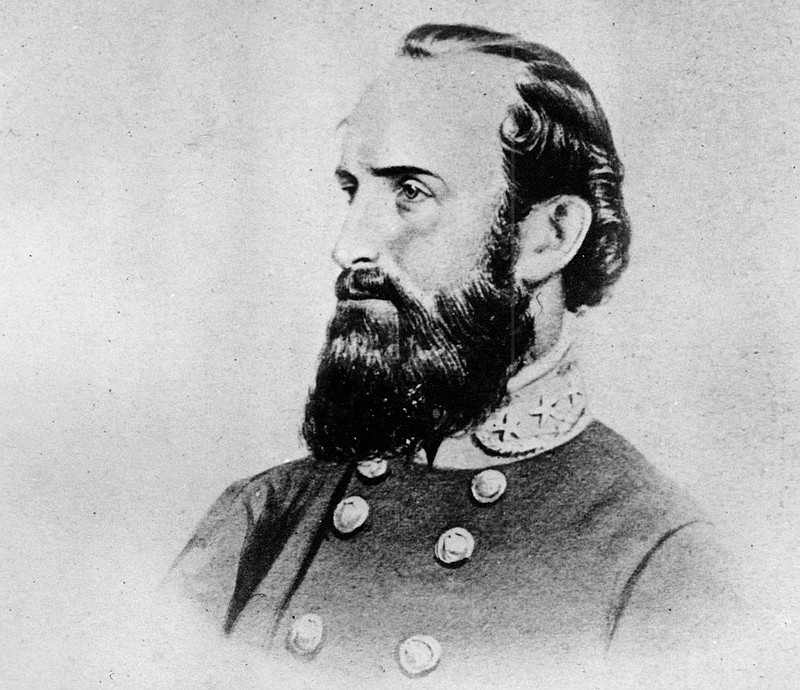In the black and white image, we see a bust portrait that stops just below the chest of a man, who is believed to be a Confederate war general, possibly Stonewall Jackson. His hair is slicked back and he has a prominent, well-trimmed long beard. His features, such as ears, nose, and eyes, are well-defined. The man is facing towards the left, providing a clear view of the left side of his face, while the right side is only partially visible. He wears a uniform with a collar, adorned with stars, and features six buttons arranged in three rows of two from the top down to the chest. The background is a solid gray with black dots, adding an aged effect to the image.